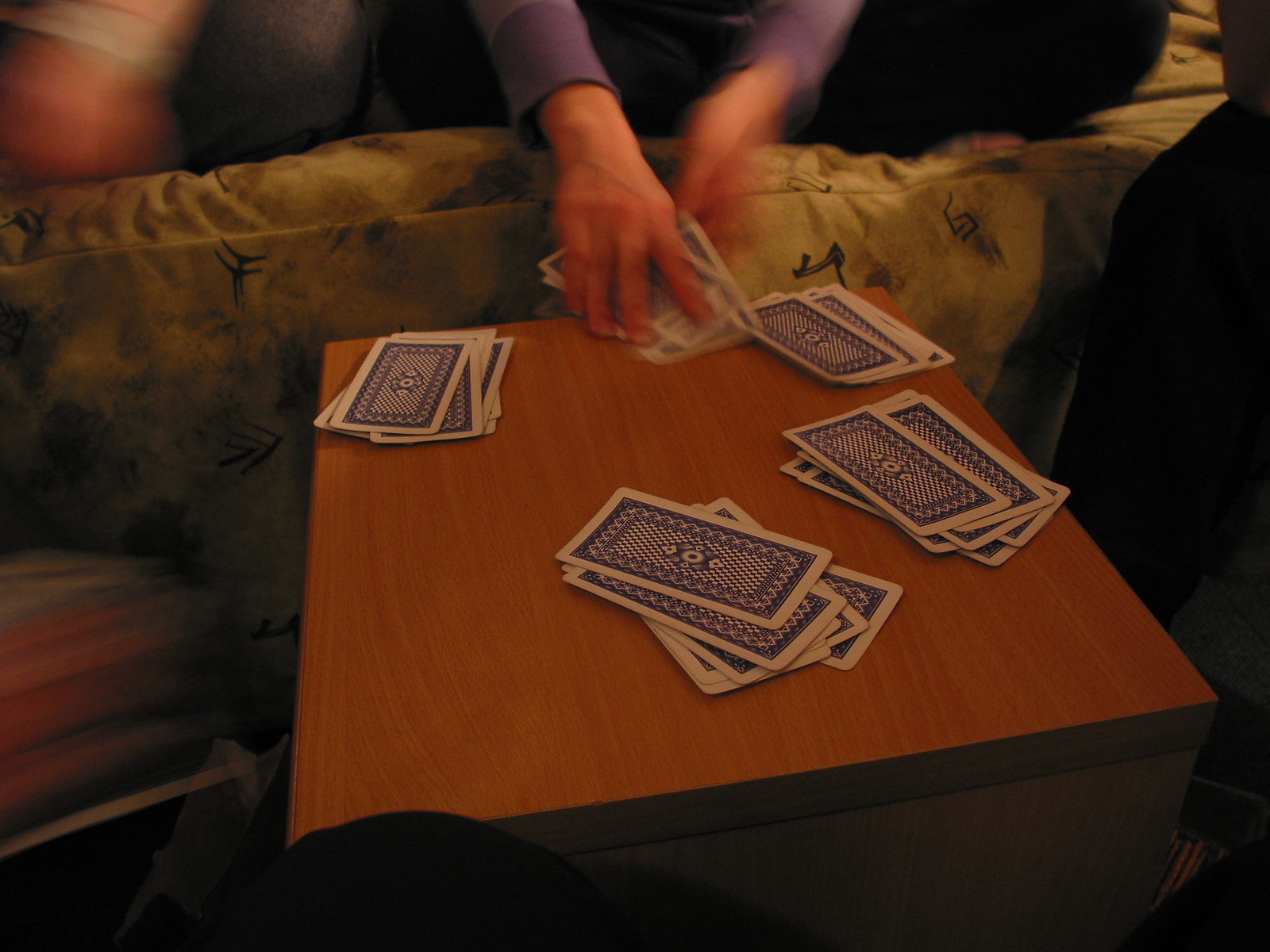In this vibrant color photograph, a person is captured in mid-motion as they kneel on a light green and brown patterned fabric slip-covered sofa. They are positioned before a low wooden table, on which five messy piles of blue and white backed playing cards are scattered. The table and cards are in sharp focus, contrasting with the slightly blurred depiction of the person, emphasizing their activity. The person's right hand is seen gripping a stack of playing cards, while their left hand appears to be reaching underneath the same stack, as if in the action of picking it up. They are wearing a long-sleeved t-shirt in a purplish-blue hue and gray or beige shorts. The photo highlights their lower arms and knees, capturing the dynamic moment in this casual and intimate setting.